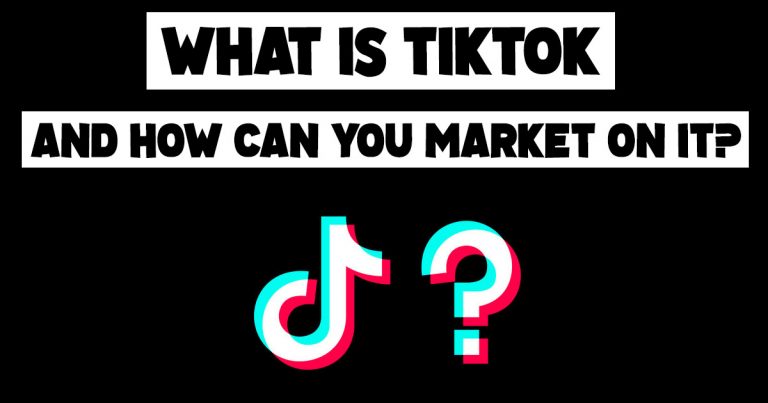The image appears to be a vertical advertisement, formatted to fit a mobile screen held horizontally. The background is entirely black, providing a stark contrast to the text elements. At the top, a white rectangle spans the center, containing the bold, black, capitalized text "WHAT IS TIKTOK". Below this, another white rectangle is present, roughly two-thirds the height of the top one. It also stretches almost the full width of the screen, stopping about a quarter of an inch from the edges. This rectangle contains the text, "AND HOW CAN YOU MARKET ON IT?" in the same bold, black, capitalized font, but in a slightly smaller size. Beneath this text, there is the TikTok logo, a blend of teal, white, and red, placed next to a question mark. This logo and question mark are also center justified and are of a very large font size, completing the visual.